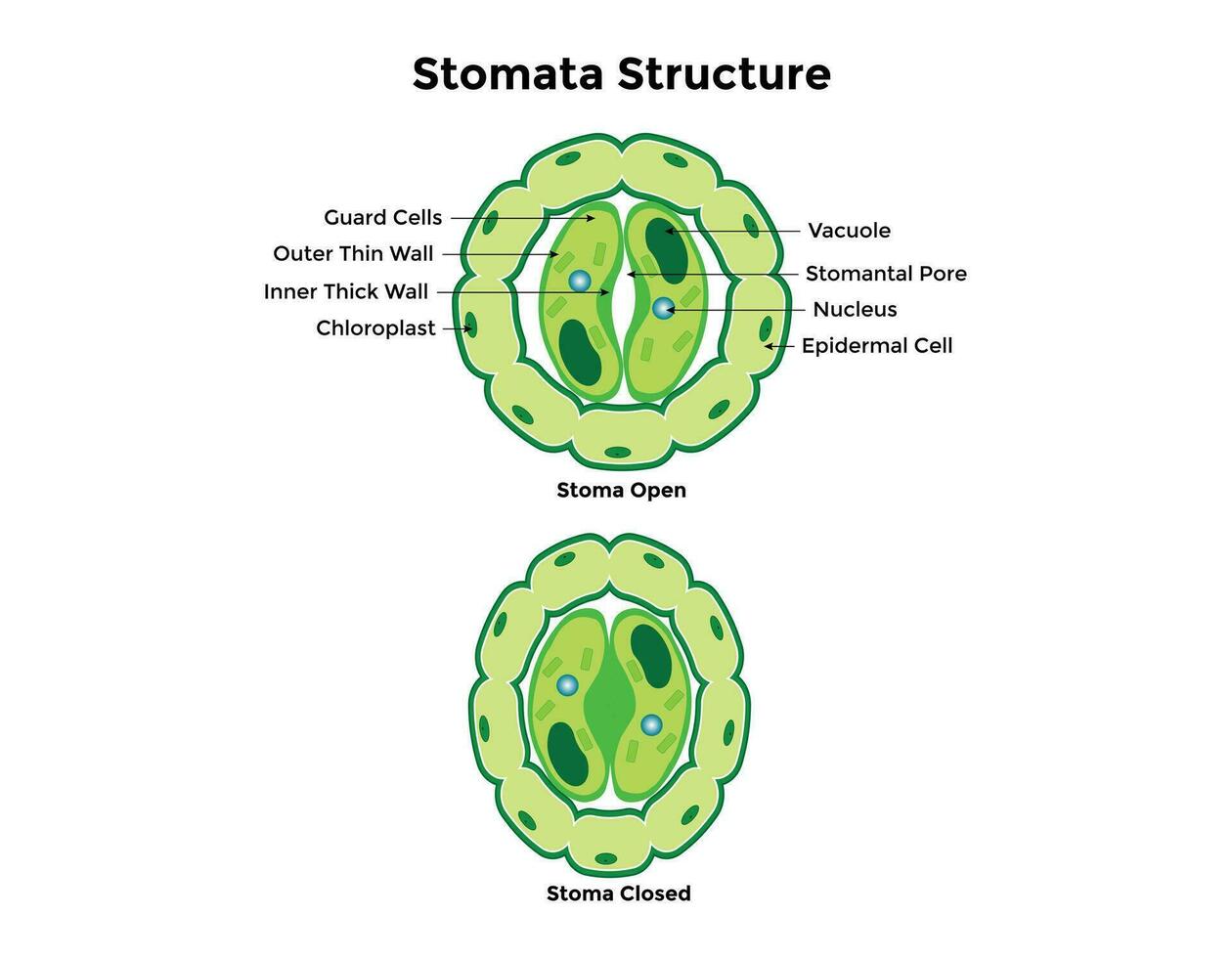The image is a detailed infographic titled "Stoma Structure," designed to support classroom or training contexts, likely in biology or botany. It features two main illustrations arranged vertically: the top illustration shows an open stoma while the bottom one depicts a closed stoma. Both illustrations are dominated by shades of light and dark green with blue spots indicating the nucleus. 

The top illustration includes comprehensive labeling of key components: guard cells, outer thin wall, inner thick wall, chloroplasts, vacuole, stomatal pore, nucleus, and epidermal cells. These labels detail the structure and anatomy of the stoma, helping viewers clearly understand the arrangement and function of each part. The bottom illustration, although unlabeled, mirrors the structural elements present in the top illustration, offering a comparative look at the stoma's closed state.

The infographic, with its green hues contrasted against a white background, is intended to give viewers a clear and organized visual representation of what an open and closed stoma looks like, making it an excellent educational tool for understanding plant cell structures.